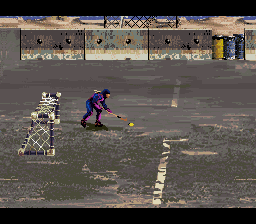In this digitally rendered image, possibly from a video game or a piece of digital artwork, we observe an outdoor skate rink. The rink's concrete surface is textured in shades of gray, taupe, and beige, adding depth and dimension to the scene. At the forefront, a hockey player stands guard in front of a goal, defending it. Captured in a side view and facing east, the player is fully equipped in a blue and purple uniform, complete with a blue helmet. The image's graininess highlights its digital nature, suggesting a moderate level of detail but not high definition. In the background, stone walls extend horizontally, framing the rink. Beyond the walls, a thin strip of what appears to be a city skyline is faintly visible, adding context and a sense of location to the scene.